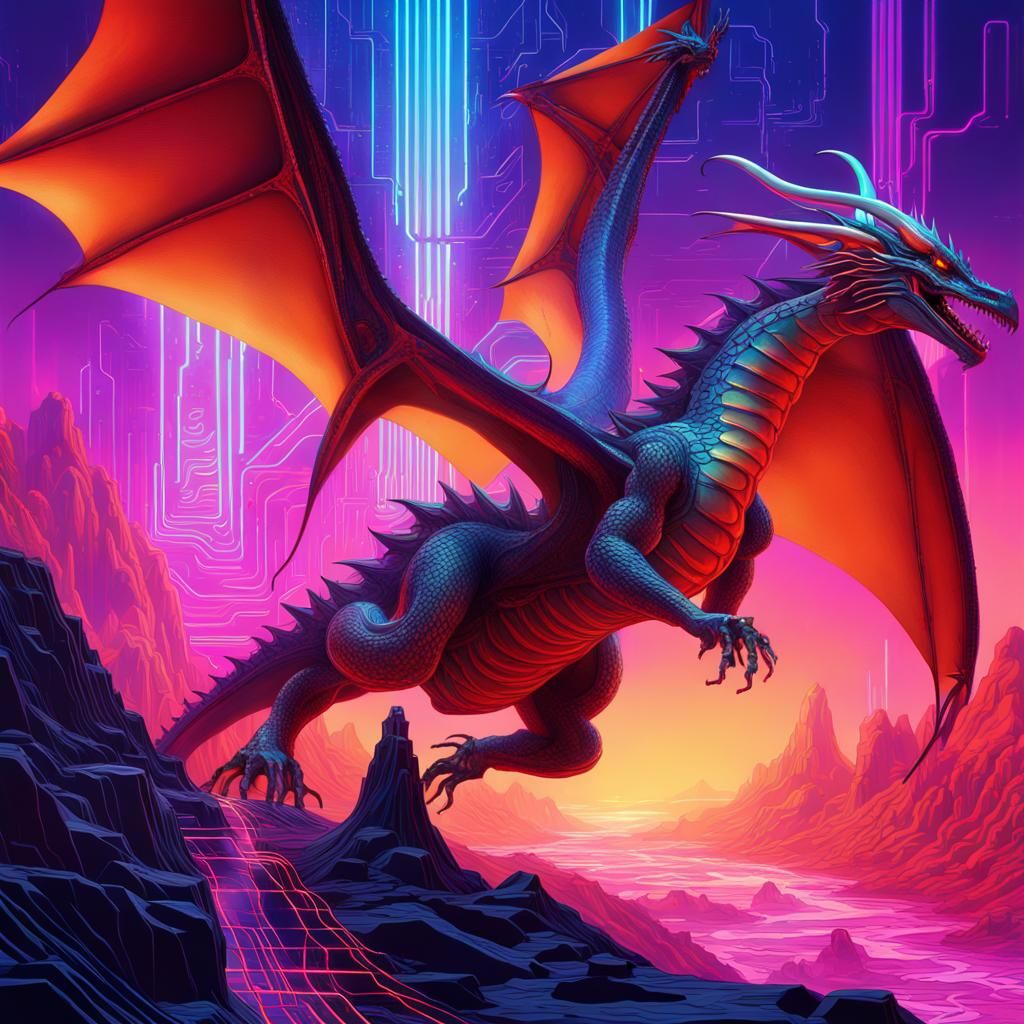This vividly colorful and modern digital art piece features a colossal dragon, dominating the entire image in a futuristic, fantasy-style landscape. The background is a surreal scene of jagged mountains with no vegetation, rendered in dark blue and pink hues, and interspersed with glowing neon lights resembling a circuit board. A peculiar pink river winds through the landscape, adding to the unearthly ambience. The dragon, poised in a powerful, ready-to-launch stance, exhibits an intense and fierce demeanor with glowing red eyes, large horns flowing back from its head, and a jagged back. Its colossal wings are brightly colored in shades of red, orange, and yellow, and the dragon’s scales display a captivating blend of blue and dark blue tones. The dragon’s muscular arms and legs are equipped with ominously long claws and seven toes each. Adding to its menacing appearance, its underbelly and teeth are blood red, and it appears ready to breathe fire at any moment. The overall tone of the painting is heavily accented by the reddish bare mountains and a mystical pink-lined path that climbs the shadowy, jagged terrain beneath the dragon's menacing right foot. The vibrant mix of colors and the intricate details of this hellish, digitalized fantasy scene make it an extraordinarily captivating piece.